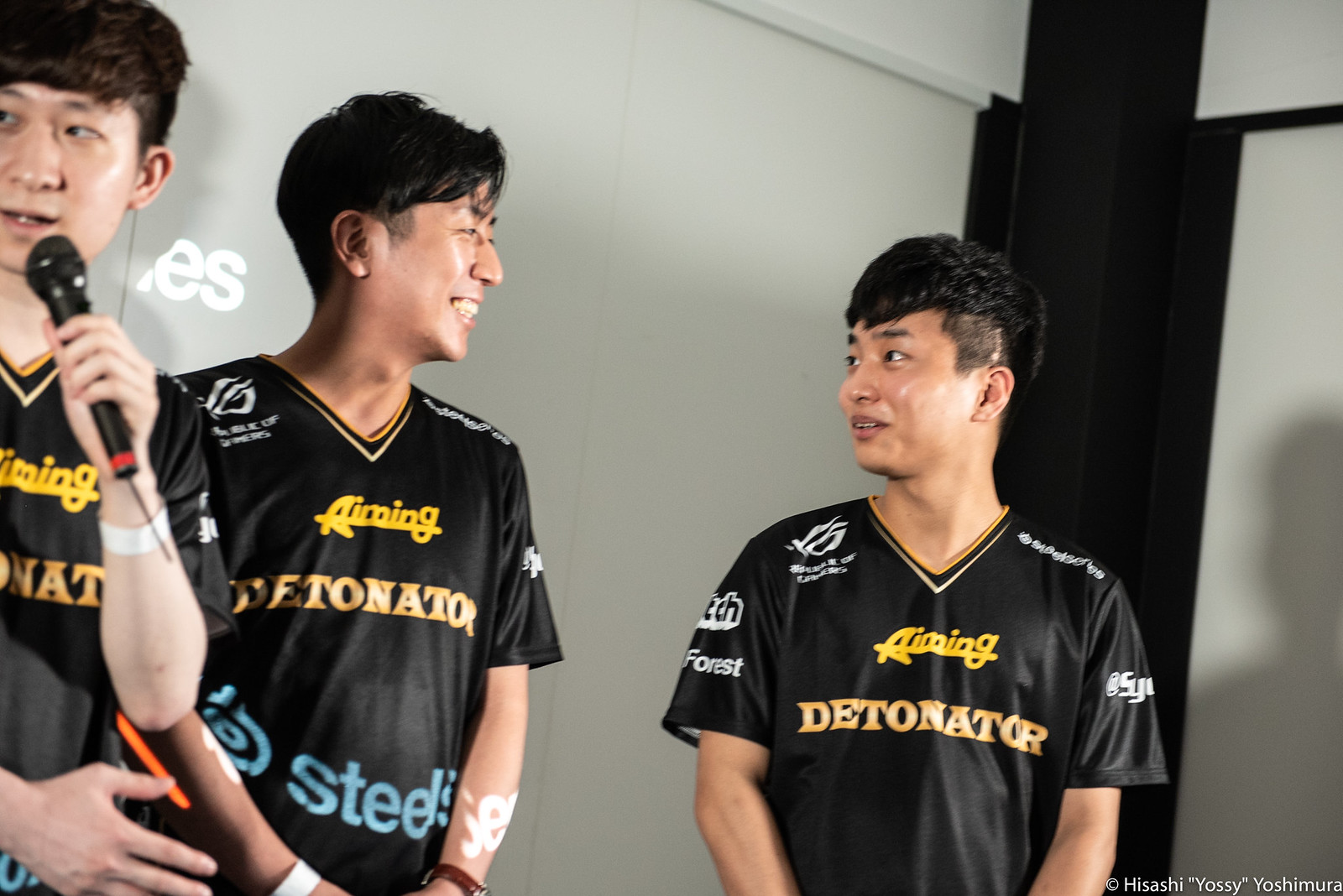The image features three Asian teenage boys, likely around 17 or 18 years old, standing against a curved white wall with a black pillar in the corner. The white wall behind them has partially visible yellow lettering that starts with "ES." All three boys have dark hair and are wearing black jerseys with various yellow and white inscriptions. The boy on the left, partially cut off, appears to be speaking into a microphone and has white tape on his left arm. His jersey, like the others, has "AIMING" at the top and "Detonator" underneath, with an inscription in blue at the bottom. The boy in the middle, who is smiling and looking at another boy, is also wearing a similar jersey and may be engaging in a presentation. The boy on the right, wearing the same black jersey, is also engaged in the conversation. Each jersey features additional text, such as "steals" in blue and "forest" in white on the right sleeve, along with an insignia in white on the right shoulder. The boys seem to be interacting closely and smiling, indicating a friendly and engaging atmosphere.